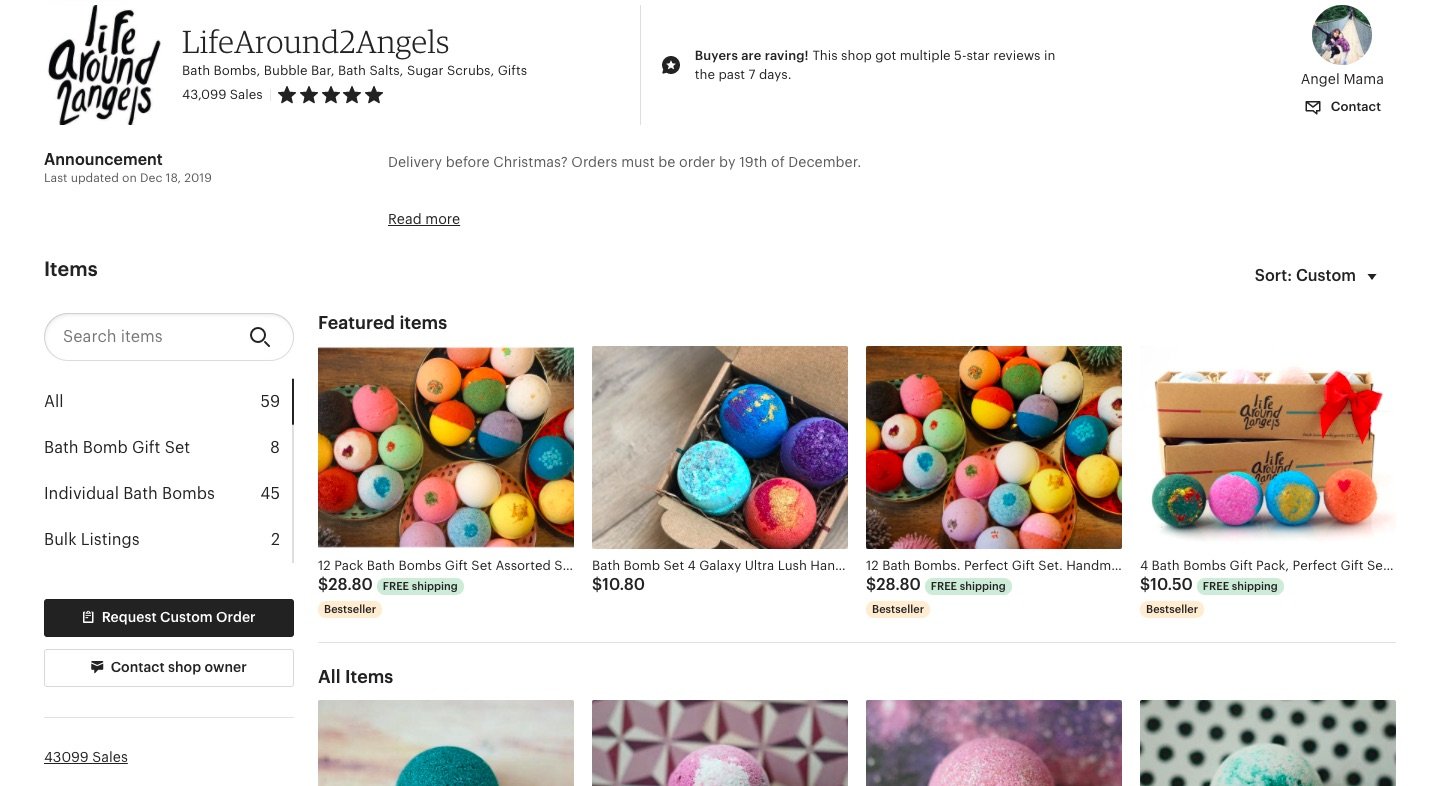This screenshot of a website page features a detailed and structured layout. In the upper left-hand corner, the title "Life Around Number Two Angels" is prominently displayed, with each word on a separate line in black text. To the right of this title, the phrase "life around the number two angels" appears in gray, running together as one continuous word. 

Below the titles are two lines of gray text, with the second line ending in a series of five filled-in black stars, indicating a rating or review. Centered on the page, black text provides further information, though the specifics are not visible in this description.

In the upper right corner, a circular profile icon features a person, though the details are indistinct. Below the icon, the name "Angel Mama" appears in black text.

On the left-hand side, approximately two rows down, a bolded black label reads "Announcement," with a line of gray text beneath it, providing more details. To the right of this, another line of gray text is present.

Further down, about four lines from the top on the left side, a section labeled "Items" is displayed, accompanied by a search bar at the top of a rectangle. This section lists various products, including "Bath Bomb Gift Set" and "Individual Bath Bombs."

On the right side, the heading "Featured Items" appears in bold black text. Below this, two rows of images showcase brightly colored bath bombs. The first row features four complete pictures, while the second row reveals the top halves of another set of four images, all highlighting the vibrant bath bombs available.